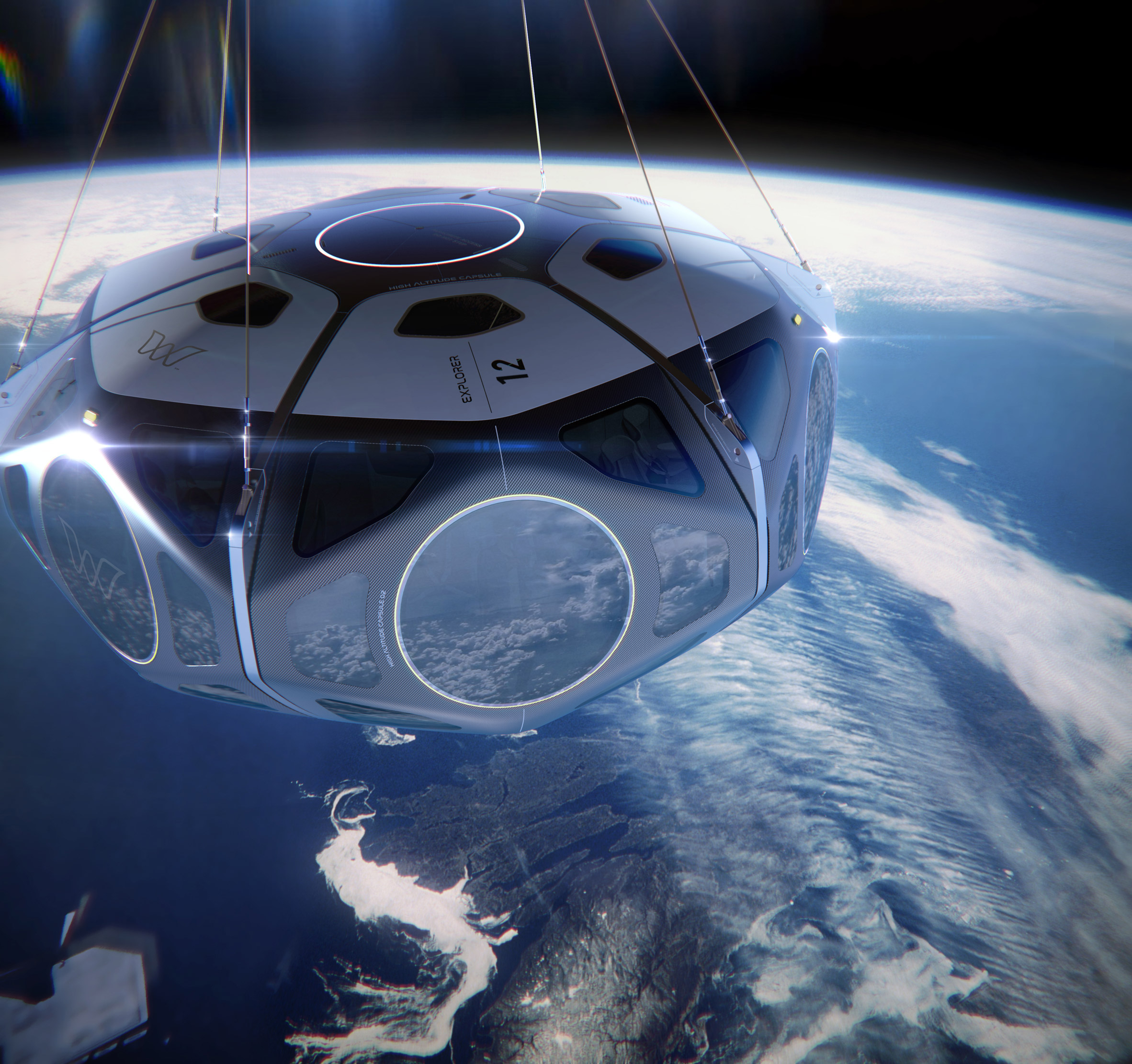The image depicts a futuristic and seemingly AI-generated spacecraft suspended high above Earth in outer space. The hexagonal-shaped craft, resembling a puffed, gusher-like structure, is connected by six steel-like cables to an unseen object above the frame. Positioned slightly off-center to the upper left corner, the spacecraft features multiple circular windows that beautifully reflect the Earth's surface below, showcasing oceans and landmasses from a great distance. Prominent text on the craft reads "EXPLORER 12," accompanied by a stylized logo that appears to be a 'W.' The image, devoid of any stars, presents a clean, detailed view of this unrealistically advanced exploration vehicle, hinting at a possible mission far beyond current technological capabilities.